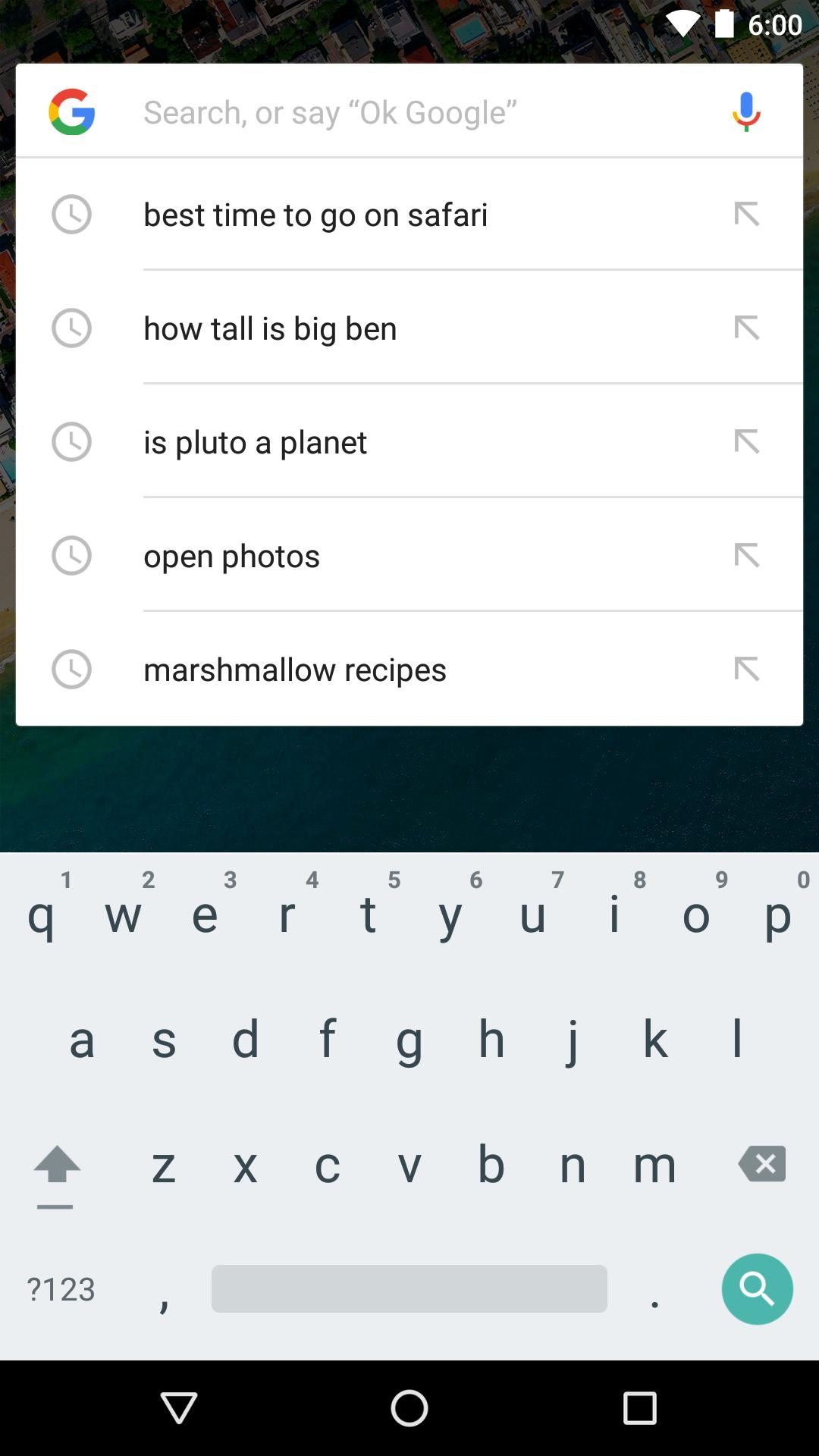The screenshot captures a cell phone screen with a black border at the top displaying icons in white for internet connection, wireless connection, and battery status. Next to these icons, the time is shown as 6:00. Directly beneath this border, a white box features the Google logo and a search bar labeled "Search or Say 'OK Google'", accompanied by a microphone icon.

Below the search bar, five suggested search phrases are listed: "Best Time to Go on Safari," "How Tall is Big Ben," "Is Pluto a Planet," "Open Photos," and "Marshmallow Recipes." Under these suggestions, an on-screen keyboard is displayed, showing letters and superimposed numbers. The keys Q to P also represent numbers 1 to 0 respectively. Additional keys include a "?123" button, a comma key, space bar, a period key, and a search key marked with a magnifying glass icon.

At the very bottom, another black border runs across the screen, featuring three white icons: a triangle pointing down on the left, a circle in the center, and a square on the right.